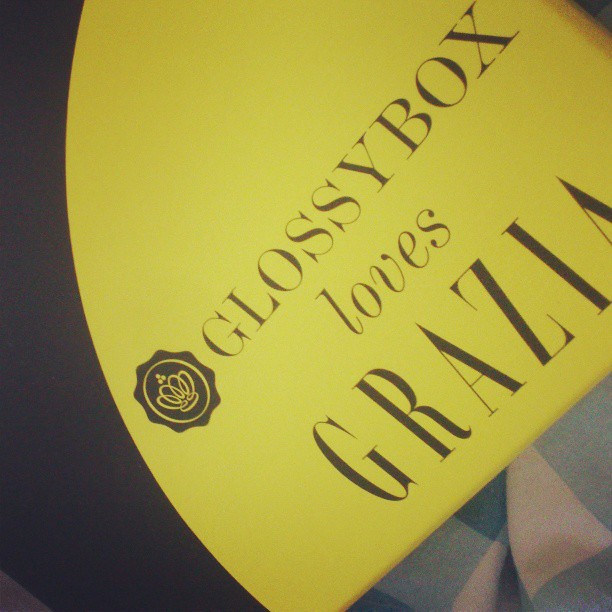The image is a detailed, full-color photograph featuring a prominently placed yellow, guitar pick-shaped sign. The sign has a background that transitions from a blue hue on the left to a lighter blue and white gradient on the lower right. This background features a subtle pattern resembling a faded creamsicle color. 

Central to the image is the main object: a bright yellow, semi-circular sign with a black print that contains three distinct types of text. Starting from the top, the first line reads "Glossybox" in elegant, dark green or black letters, placed to the left of a black emblem. This emblem showcases a yellow circle with a crown comprising three smaller circles above it. Below "Glossybox," the word "loves" is written in cursive script, and beneath it, the letters "G-R-A-Z-I-A" can be discerned, although the full word appears slightly obscured or cut off, implying it spells "Grazia."

The photograph is taken at an angle, which possibly displays part of the corner of a box, indicated by the partial view and the slight distance visible in the lower right corner. The overall ambiance suggests that the sign may be part of a setting inside a building, possibly related to a corporate or retail environment associated with the "Glossybox loves Grazia" branding.